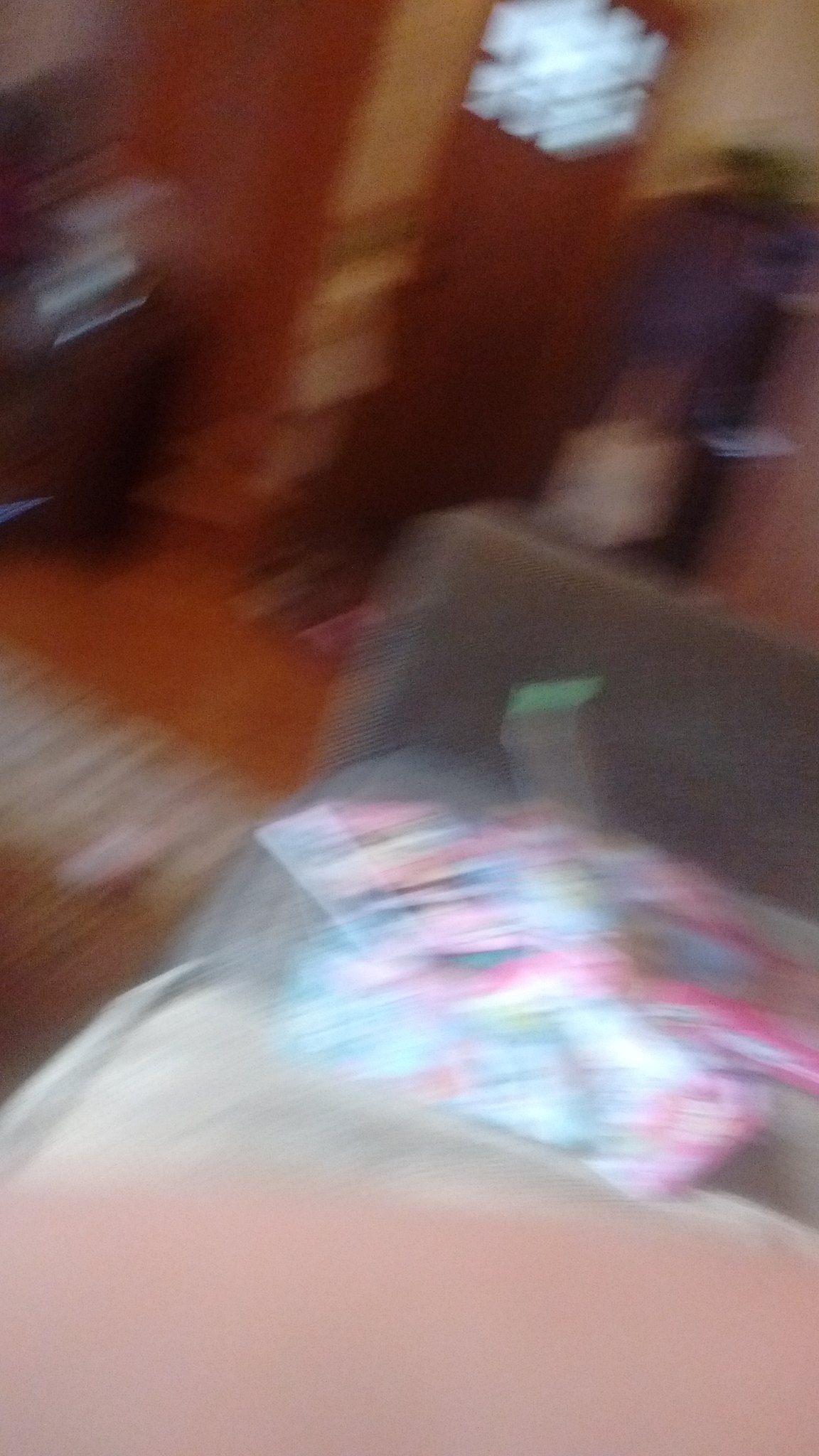This vertical, blurry photograph features the interior of a living room with a modern taupe-colored couch as its main focus. The image appears to be partially obscured by what seems to be a person's finger over the lens at the bottom, contributing to an almost double exposure effect. The couch hosts indistinct, blurred objects that resemble an upside-down table or stand. Adjacent to the couch, a doorway framed in a lighter color is visible, showcasing a multi-paneled window allowing light to filter through. Before the doorway lies a planter with vivid purple foliage. On the floor, a rug marks the entrance to the living room, complemented by another area rug positioned in front of the couch. In the upper left corner, a possibly black television or stereo components can also be faintly observed.